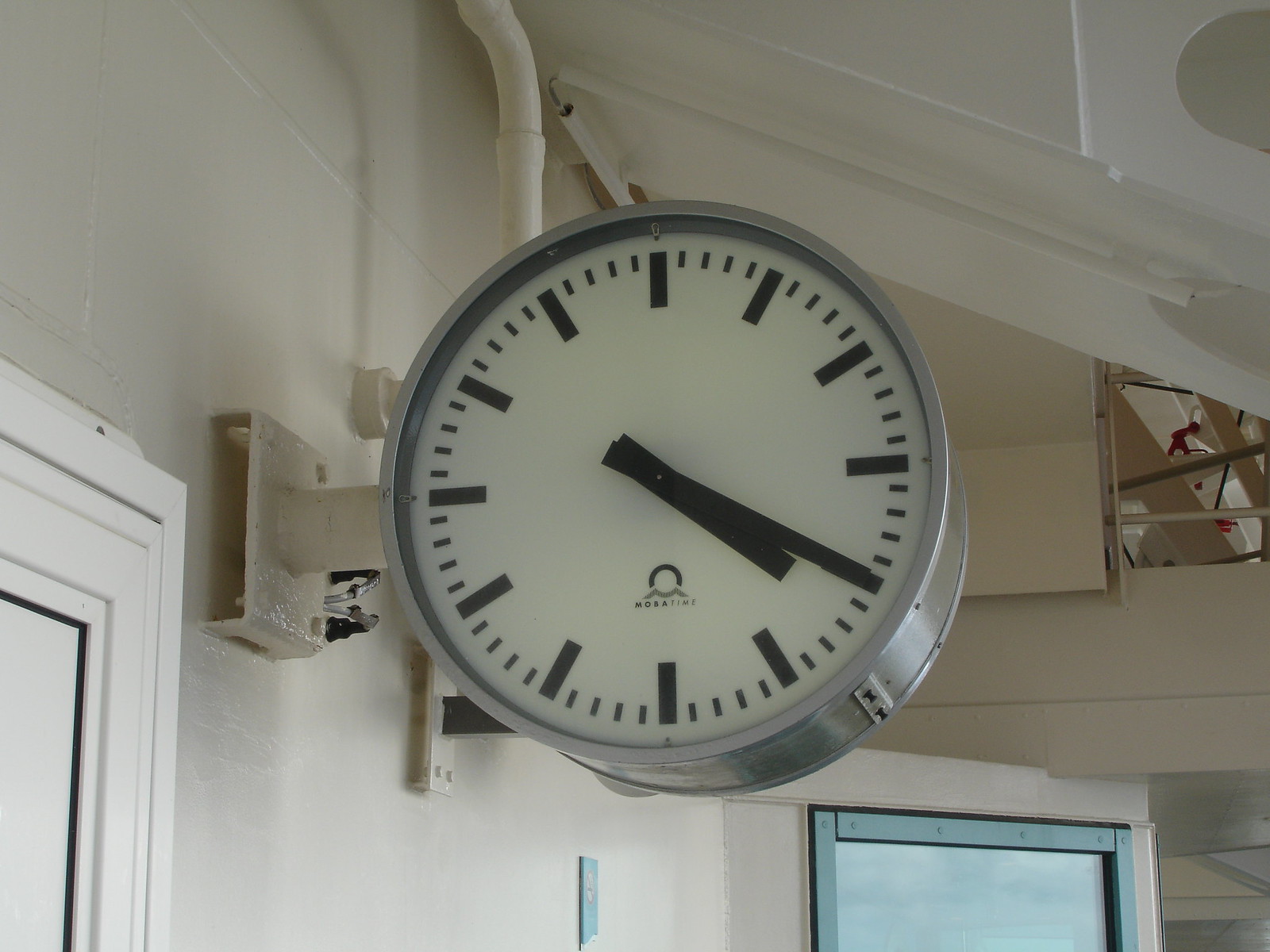This image features a large, silver-rimmed clock mounted on a beige wall, possibly in a commercial or public space like a train station. The clock, attached to a metal pole protruding from the wall, is designed to be visible from both sides. Its face is white and minimalist, adorned with bold black hour and minute markers, and thick black hands, though it lacks a second hand. The manufacturer's logo, which reads "MOBA time," sits at the bottom center of the clock face, accompanied by a small emblem above the text. Around the clock, the building's infrastructure is visible, including steel girders, ductwork, and piping, all painted a very light beige. To the left of the clock is the corner of a white door, and to the right is what appears to be a black-framed doorway, though the image cuts off, making the exact nature of the right-side entrance unclear.